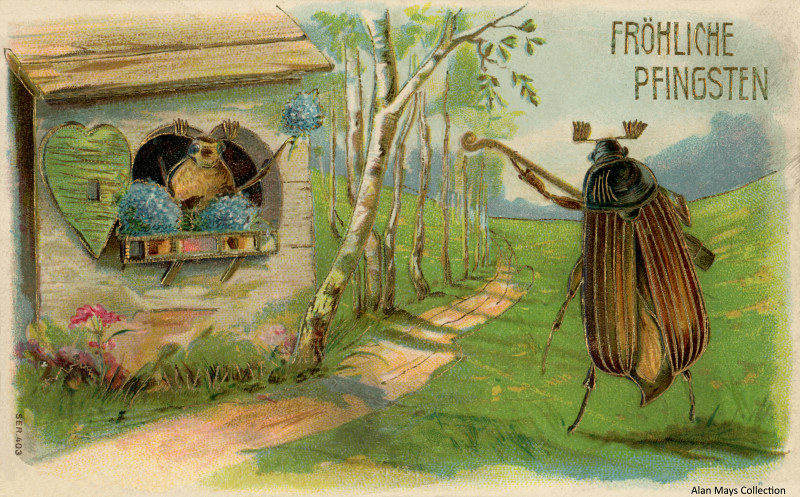This detailed and graphically created artwork, likely done in paint on old beige-toned paper, presents a whimsical scene entitled "Fröhliche Pfingsten" (Merry Pentecost) as noted in the sky of the image. The drawing depicts a cricket or a beetle holding a musical instrument, resembling a guitar, walking along a winding path lined with tall trees with white trunks. On the left side of the path is a small shed-like home, from which another insect peeks out through a window, holding a bouquet of flowers. The insect inside the home appears to be engaging with the musical performance outside. The image is thoughtfully composed, evoking a quaint and festive atmosphere. This piece belongs to the Alan May collection.